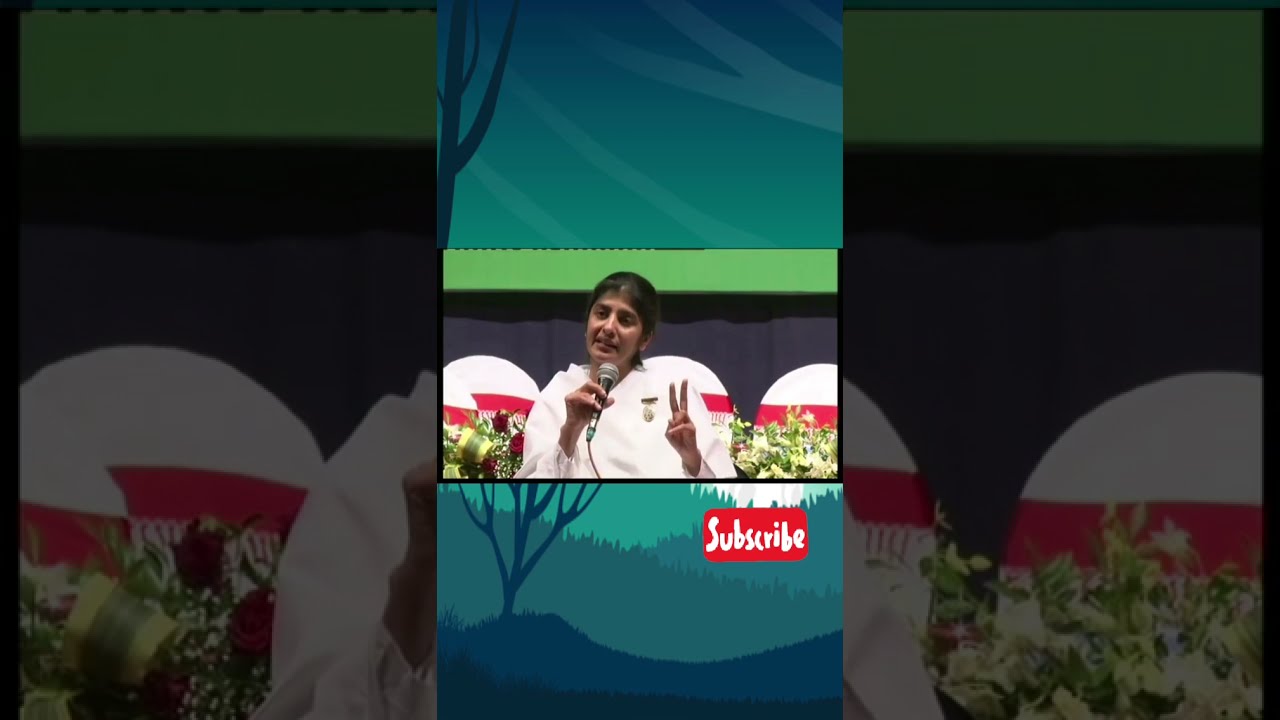The photorealistic image features a South Asian woman with dark black hair, wearing a white shirt, standing at the center while holding a microphone in her right hand and giving a peace sign with her left hand. She has a slight tilt to her head and her hair frames her face. She is surrounded by seating that is white and red in color, and there are bouquets of flowers with green leaves, white, and red flowers nearby. The central image, which takes up the middle third of the screen, is flanked on both sides by darker, zoomed-in sections of the same photograph. Behind her is a background featuring a green stripe at the top, a black line underneath, and a gray section that disappears behind the chairs and flowers. Above this setup is a computer-generated design with a gradient turquoise color scheme, displaying silhouetted trees and plants, including dark blue trees. A red subscribe button with white text is prominently displayed within this stylized design.